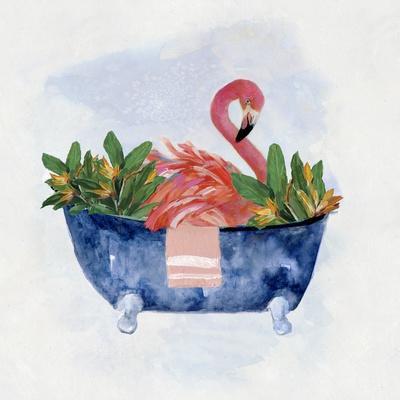The image depicts a flamingo with distinct pink hues, both light and dark, sitting in a historical clawfoot bathtub which is a bluish-white color. The flamingo's neck is gracefully curved downwards, and its black and white beak is visible. Its feathers jut out prominently. The bathtub is adorned with a tan and white striped towel (or possibly pink as suggested by one description) draped over the front edge. Surrounding the bathtub are plentiful green leaves, interspersed with hints of yellow leaves or flowers, adding a touch of natural beauty. The background features a very light blue and white color scheme, lending a subtle airy feel to the scene. The illustration, capturing a whimsical moment, seems to be rendered in a medium reminiscent of watercolors or colored pencils, and it definitively lacks any text or signature. The overall dimension of the image is a perfect little square.